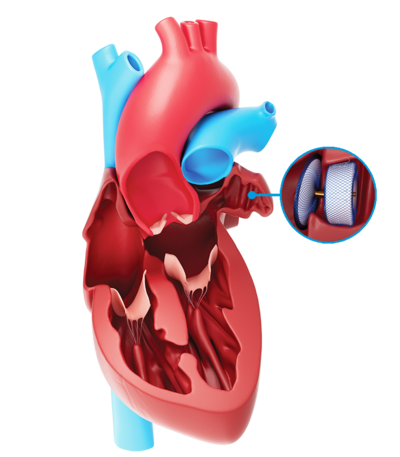In this detailed medical illustration of a heart, we see a plastic-like, cartoony render of the organ dissected to showcase its interior. The heart is predominantly colored in shades of light red and orange, with the upper section in a lighter red hue and featuring three open valves. Surrounding the structure, there are areas with darker red hues and some flame-like patterns, representing arteries and veins. 

Prominently, there's a circular section on the right, connected by a blue line that points to the heart. This circle zooms in on a medical device, which appears to be a stent or filter. The device consists of a ring-like structure with a metal tube, or pipe, passing through it, alongside a disc-shaped component of similar material. Both parts are crafted from a white mesh with blue lining around the edges. 

The overall background is white, making the colored sections stand out. The blue areas specifically highlight certain arteries and veins, emphasizing the location for potential medical device placement.